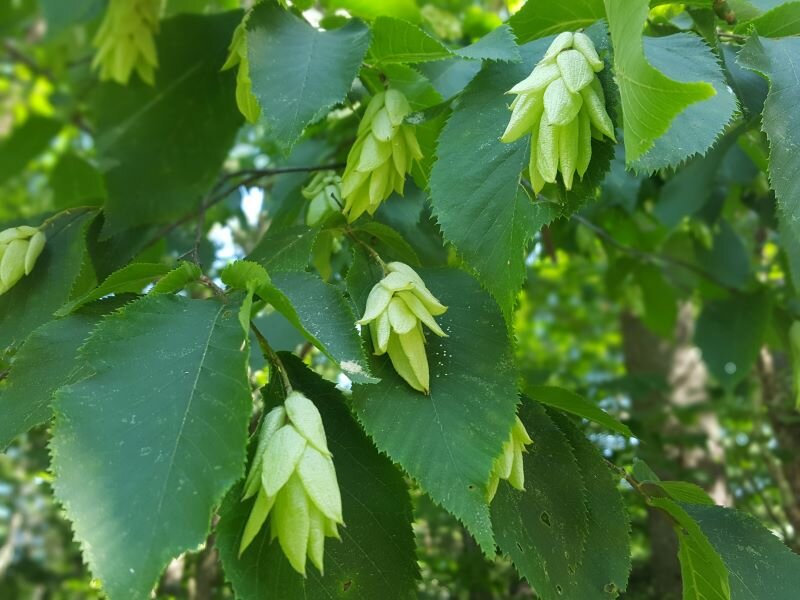This photograph captures a close-up view of the leaves and budding seed pods on a tree, taken outdoors during daytime. The image prominently features a variety of greens, ranging from dark green large leaves to smaller, lighter green leaves clustered together, creating a vibrant and lush composition. The large leaves are elongated, elliptical, and feature prominent central veins with diagonal veins branching out towards their spiked edges, while the undersides of these leaves reveal a brighter, lighter green when they curl.

Additionally, the photograph showcases small, light green clusters that appear to be seed pods or new buds emerging from the ends of thin branches. These clusters are initially in pairs and multiply as they progress, rotating around the branch tips. The few visible thin branches supporting the foliage are dark in color. Bright sunlight filters through the leaves, casting shades of green throughout the photograph, with specks of white on some of the leaves adding texture and depth.

Despite being a close-up shot that focuses on the details of the leaves and pods, the background subtly reveals hints of a wider outdoor setting, where the white and blue sky peeks through the gaps in foliage, providing a glimpse of the broader environment.